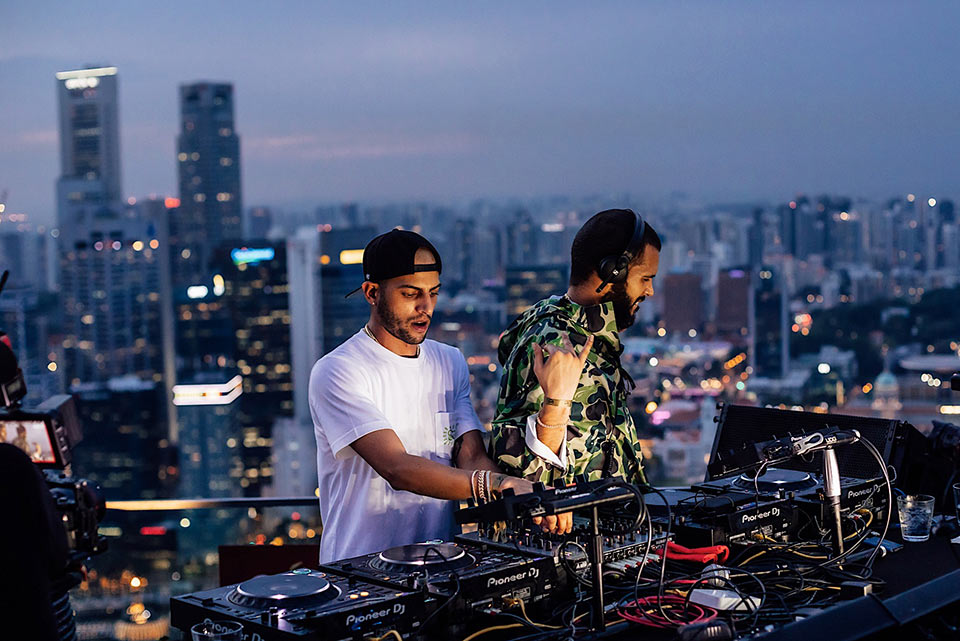At dusk, on a rooftop in a bustling metropolitan city, possibly New York City, two DJs are setting the stage for an anticipated rooftop party. The air is filled with the electric ambiance of early evening, as dim city lights begin to twinkle against a backdrop of gray and white clouds. The rooftop is adorned with intricate DJ equipment, the wiring meticulously set up for two performers. One DJ, wearing a black hat backwards, a white t-shirt, and several bracelets, is intensely focused on adjusting the knobs and switches. This DJ also sports a short beard and an open-mouthed look of concentration. The other DJ, donning headphones and a camouflage jacket, has a thicker beard and raises one hand in an animated gesture, possibly dancing. He is slightly darker-skinned and also wears several bracelets. Behind them, a camera crew captures both the scene and the DJs, while the vast, dense array of skyscrapers in the city's skyline lights up as night falls.